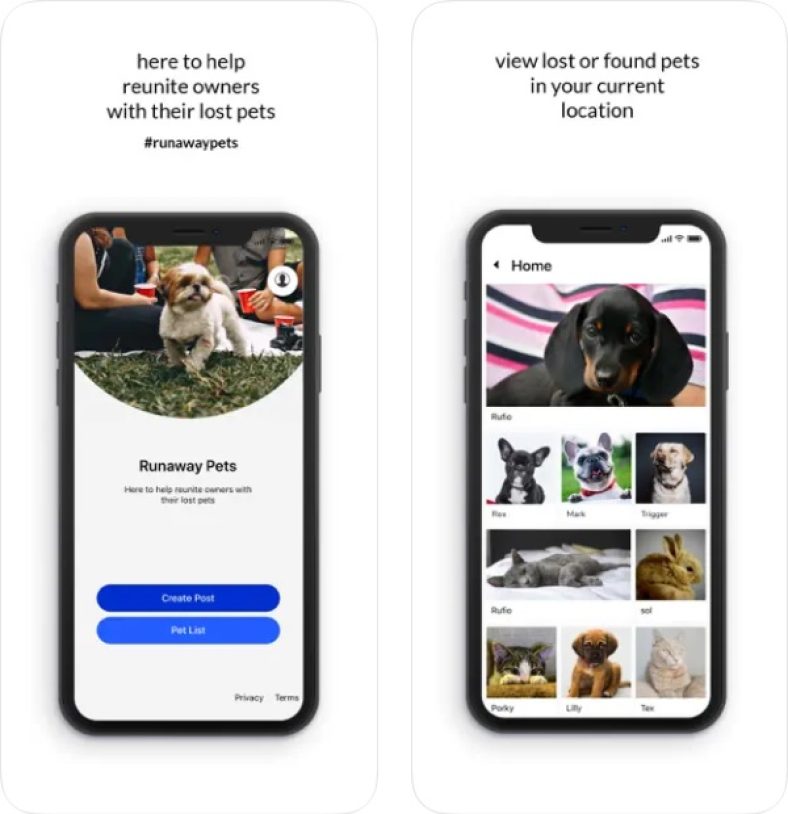This screenshot likely comes from a webpage or display ad designed to aid in the reunification of lost pets with their owners. The image consists of two smartphone screenshots placed side by side, each encapsulated within a very thin grey line against a white background.

**Left Screenshot:**
- **Headline:** In all lowercase grey font, the headline reads, "here to help reunite owners with their lost pets."
- **Subtitle:** Below the headline, a hashtag reads "#runawaypets."
- **Smartphone Display:** 
    - **Image:** A photo of a small, shaggy-haired dog with a white body and brown fur around its ears. The dog is standing on grass, accompanied by the torsos of a couple of people sitting nearby.
    - **Text:** A repeated phrase, "runaway pets," followed by, "here to help reunite owners with their lost pets."
    - **Buttons:** Below the text are two buttons. The top button, in royal blue with white font, says "create post." The second button, in sky blue, has text that is too small to read.

**Right Screenshot:**
- **Headline:** In all lowercase grey font, it reads, "view lost or found pets in your current location."
- **Smartphone Display:**
    - **Image:** Features several animal photos. 
        - **Top Photo:** A close-up of a dog with predominantly black fur and some brown around the nose.
        - **Rows of Photos:**
            - **Top Row:** Three photos, each of different dogs.
            - **Middle Row:** Two photos, one of a cat and another of a rabbit.
            - **Bottom Row:** Three photos, including a kitten, a puppy, and an unidentified white animal, possibly a cat.

This descriptive caption offers a detailed breakdown of the screenshot, highlighting key visual and textual elements to provide a comprehensive understanding of its content.